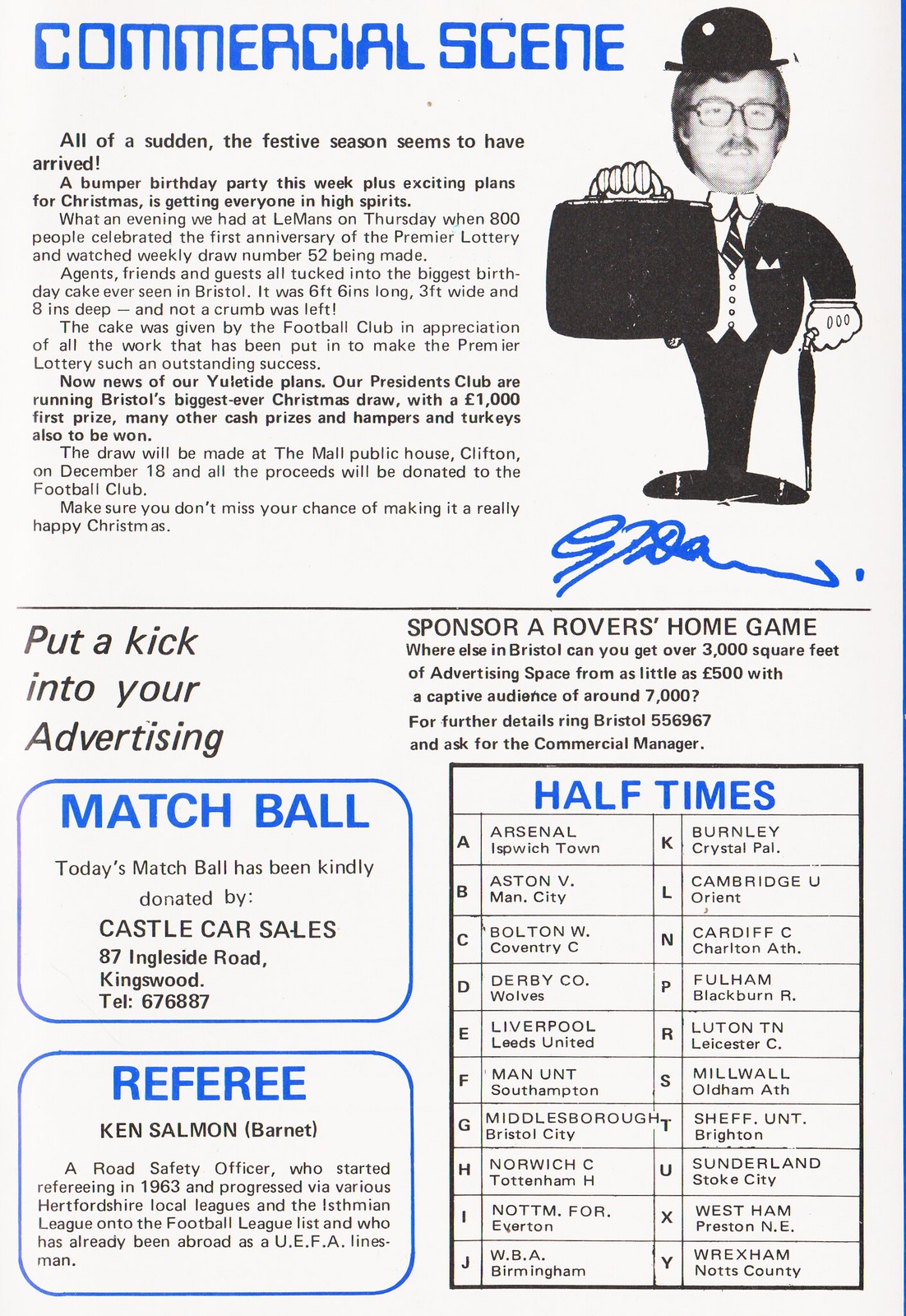The advertisement, designed in a vintage 80s computer-style font, features a striking photograph of a gentleman in a tuxedo, blending an actual photo of a man's head with cartoonish elements. It announces, "All of a sudden, the festive season seems to have arrived," highlighting how a bumper birthday party this week and exciting Christmas plans have put everyone in high spirits. The text, primarily in black with blue accents, further describes a memorable evening at Le Morte, where 800 guests gathered for the first anniversary of the premier lottery and the 52nd weekly draw. They celebrated with the largest birthday cake ever seen in Bristol, gifted by the football club in gratitude for the lottery's success. The bottom of the advertisement informs readers on how to invigorate their advertising by sponsoring a Rovers home game, referencing aspects like matchballs, halftimes, and referees—indicating it might be from a program for the Rovers, a local sports team.